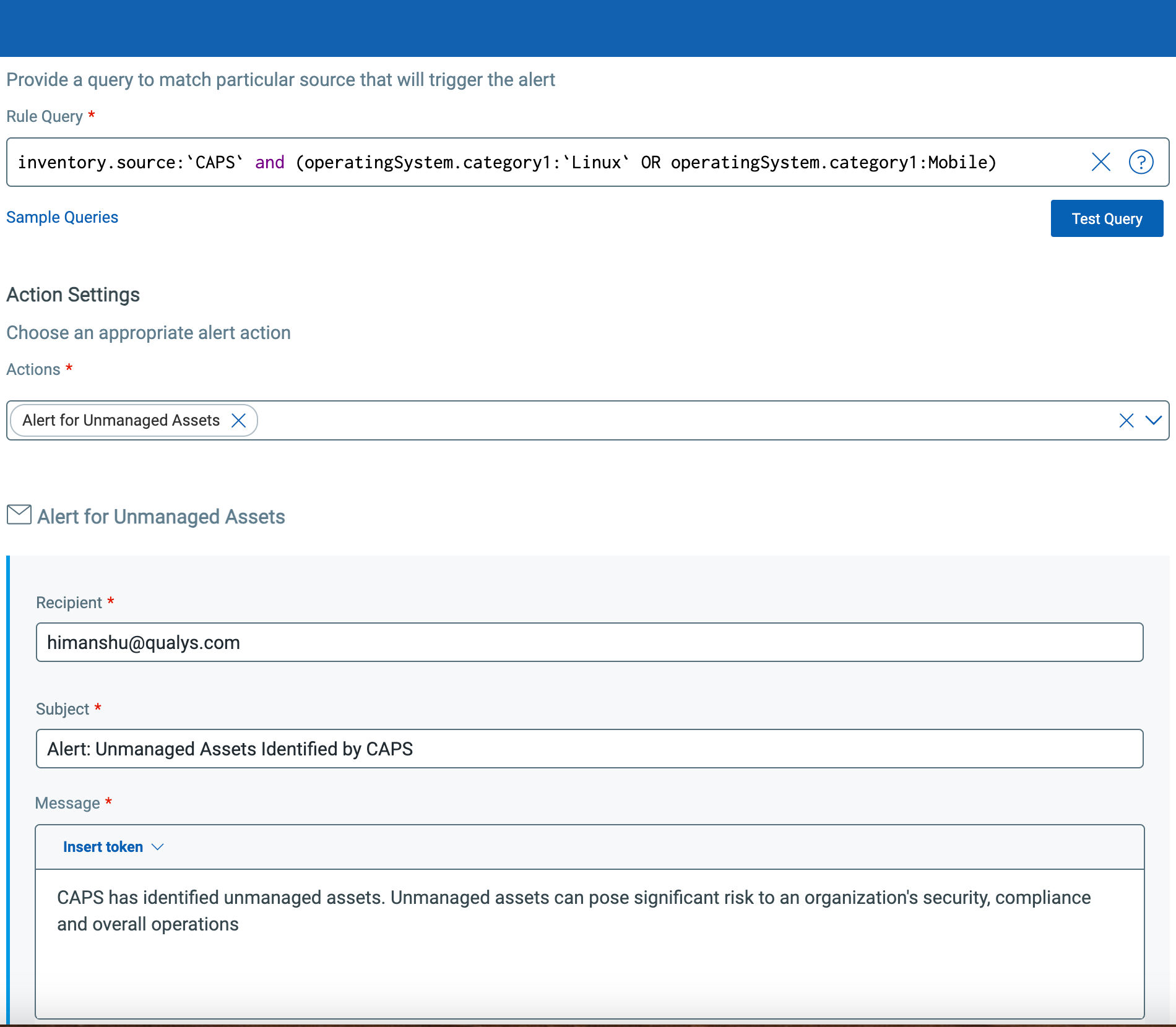A screenshot captures a software interface displayed against a white background. At the very top, a small blue bar, devoid of text, crowns the page. Just below this blue bar, in small blue font, is an instruction: "Provide a query to match a particular source that will trigger the alert." Directly beneath, aligned horizontally from left to right, the text "Rule Query" is present, accompanied by a red asterisk, indicating a required field. In an adjacent search bar, a rule query has been input by the user.

Further down and to the left, there is a hyperlink labeled "Sample Queries." To the right of this link, a button labeled "Test the Query" is available for validating the input.

The subsequent section is titled "Action Settings" with the directive "Choose an appropriate alert action." Following this, "Actions" is marked with a red asterisk, signifying another mandatory field. A dropdown menu is provided for the user to select the relevant alert actions.

Continuing downward, a small mail icon is displayed next to the text "Alert for Unmanaged Assets." Below this, the label "Recipient" with another red asterisk denotes a required email input field. Users can type in the recipient's email address here. Beneath that, the field "Subject," also marked with a red asterisk, prompts users to type in the subject of the alert email. Lastly, a text box is available where users can enter their message content. An example message has already been typed into this field.